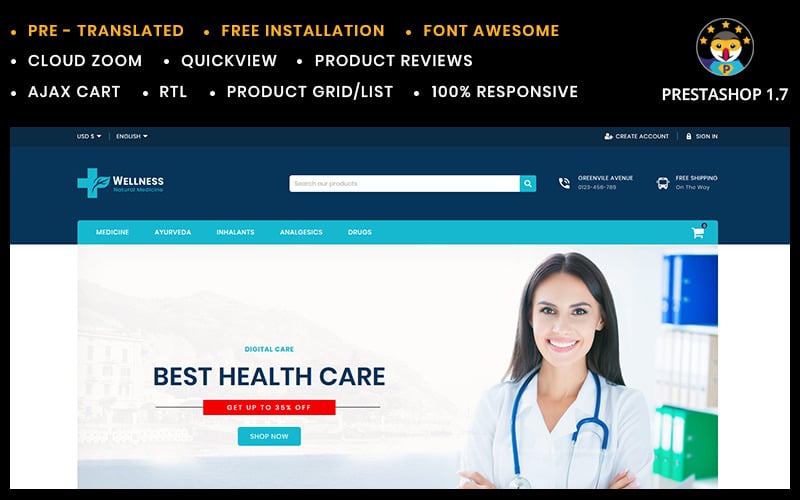This image is a detailed screenshot showcasing different elements of an e-commerce webpage. At the top, in a banner-like format, various features are listed: Pre-Translated, Free Installation, Font Awesome, Cloud Zoom, Quick View, Product Reviews, AJAX Cart, RTL, Product Grid/List, and 100% Responsive. 

To the right part of the image, there is a vibrant cartoon illustration of a superhero character. The character is depicted wearing a yellow mask over their eyes, with a curved line of yellow stars arching behind their head. They appear to be clad in a classic superhero uniform.

Below this section, there is a navigation bar with links and options such as PrestaShop 1.7, US Dollars, English, Create Account, and Sign In. Adjacent to these options is a prominent blue cross symbol, under which is the text: Wellness, Natural Medicine. Furthermore, it includes a search bar with placeholder text "Search our products" and contact details listed as Greenville Avenue, 0123-456-789.

The webpage also promotes several categories and offers: Free Shipping On The Way, Medicine, Ayurveda, Inhalants, Analgesics, and Drugs. A shopping cart icon is present, followed by promotional messages: Digital Care, Best Healthcare, Get Up To 35% Off, Get Up Now.

Dominating the right side of the frame is a photograph of a young, fair-skinned woman with long dark hair parted in the middle. She is directly facing the camera with a warm smile. The woman is dressed in a white lab coat, and a blue stethoscope is draped around her neck. She stands with her arms crossed over her chest. The background includes a bookshelf filled with blue, white, and green books, giving a sense of a professional and well-organized medical setting. The overall dimensions of the image are wider than it is tall, providing a clear, expansive view of the content.